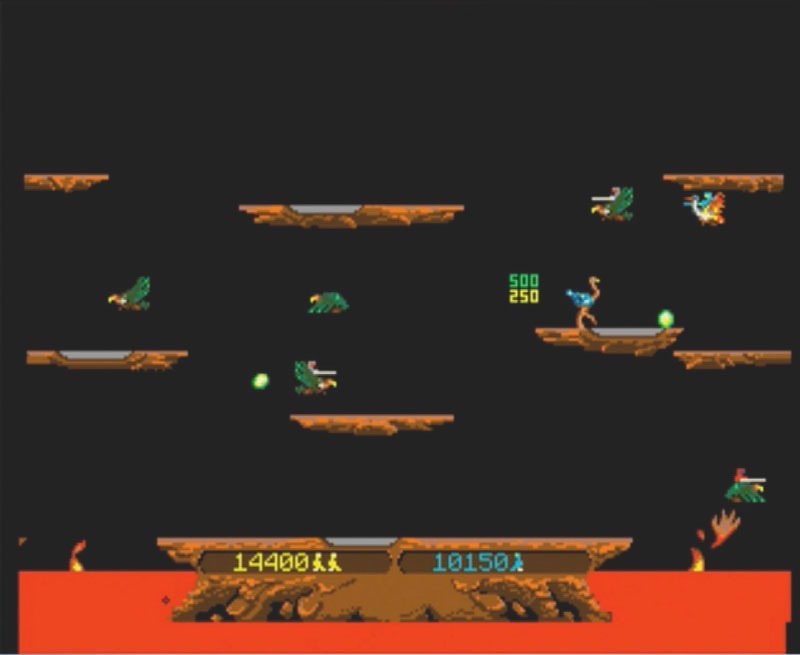The image depicts a vintage screen from the classic 1980s arcade game "Joust." The gameplay area is structured with several platforms suspended above a sea of bubbling lava at the bottom of the screen. There are numerous floating platforms: one in the middle, a pair towards the right, with one positioned higher above the other, another to the left, and higher platforms symmetrically spread throughout the screen.

The left player’s score is prominently displayed in yellow as 14,400, with two lives remaining. Meanwhile, the right player's score is 10,150, shown in blue, with only one life left. The characters, mounted on ostriches, navigate these platforms. Specifically, one ostrich is seen landing on a lower right platform, approaching a glowing egg. The screen is busy with action; six green buzzards fly erratically across the stage, adding to the chaotic battle environment.

Two numerical tags float in the scene: "500" in green situated behind the ostrich and "250" in yellow just below. These likely represent bonus points for collecting the glowing eggs or defeating enemies. The game’s nostalgic 1980s graphics and the frenetic pace are captured clearly, evoking a sense of excitement and childhood memories for those familiar with this iconic arcade game. The game is unmistakably identified as "Joust," a beloved title from the era that brilliantly encapsulates two-player cooperative or competitive gameplay.